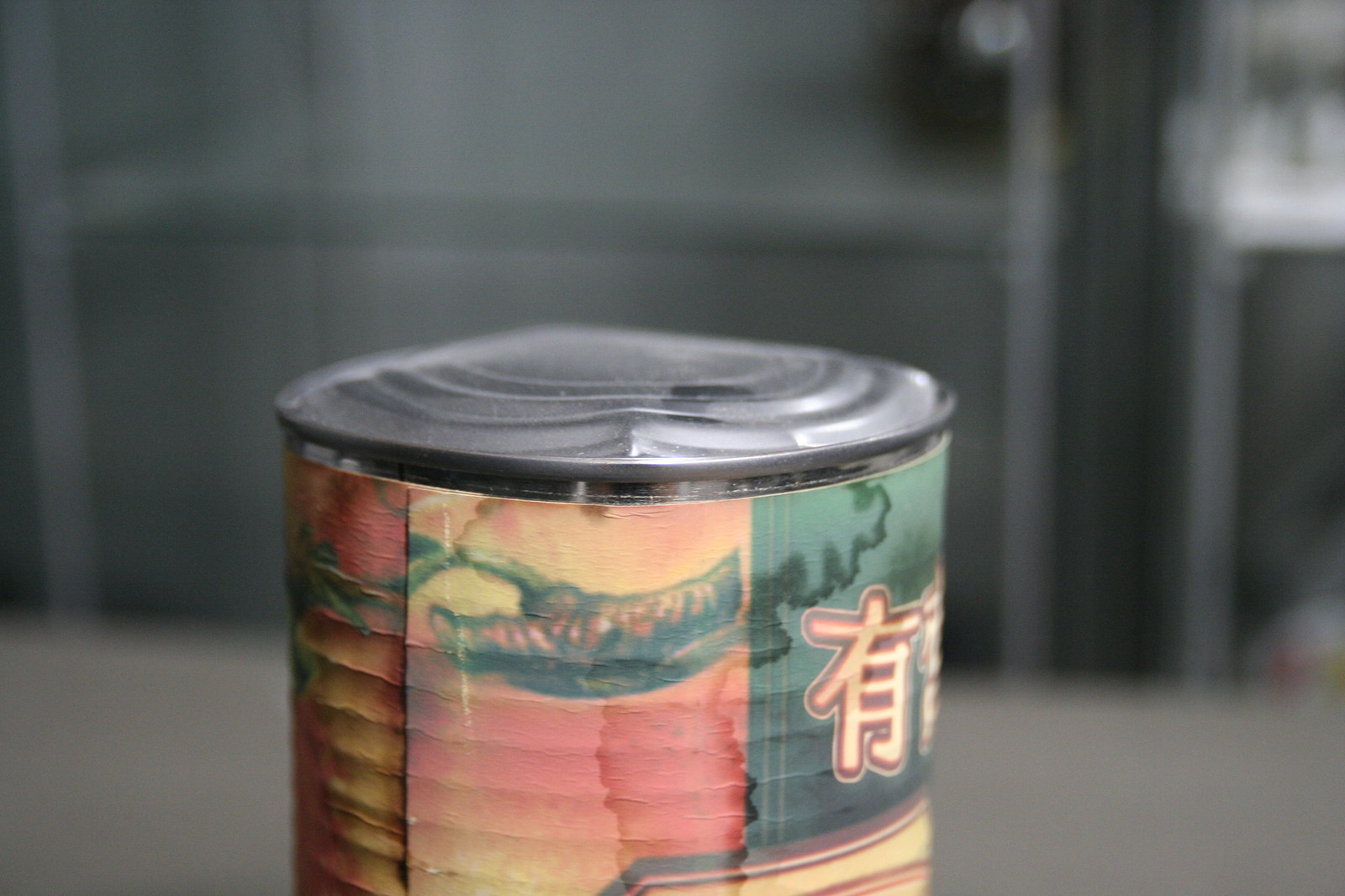This image captures a somewhat battered can, prominently featured in the foreground with an out-of-focus background that hints at a kitchen setting—perhaps with shelves, a door, or a counter. The can itself, showing signs of heavy wear and tear, has a slightly bulging and dented top, with a jagged edge suggesting it has been struck hard enough to cause minor separation from the body. The multicolored label—bearing what appears to be Chinese or Japanese characters—wraps around the can, displaying hues of red, yellow, green, and peach, and possibly depicting illustrations of chilies or other plants. The label appears stained and aged, with watery marks and ribbing visible underneath, indicating it may have been sitting for a very long time.